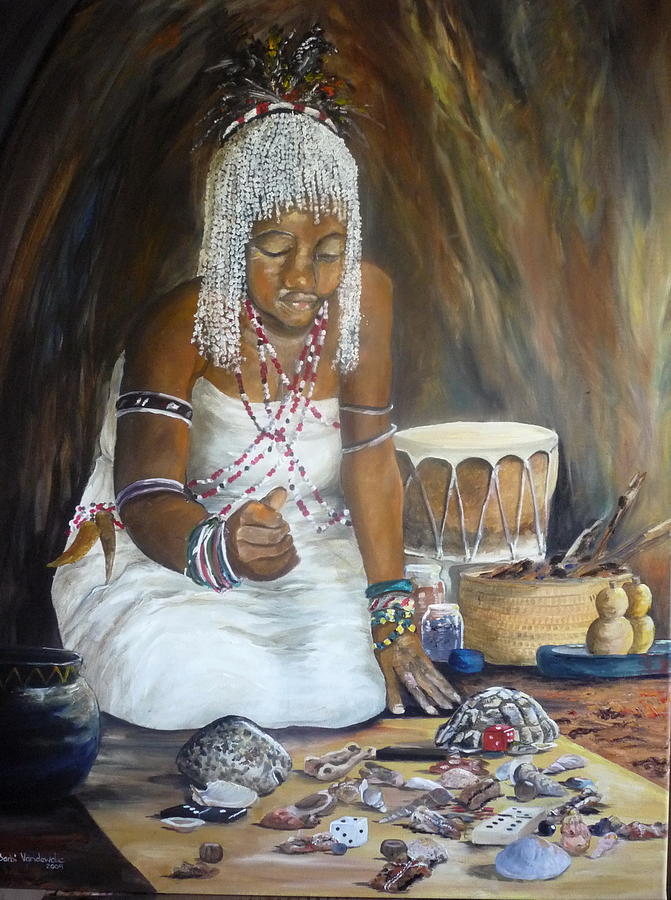The vertically oriented painting depicts an African or Native American woman with dark skin inside what appears to be a cave or hut, characterized by a background of various shades of brown, yellow, and gray brushstrokes. The central figure, a young woman or teenage girl, is adorned with a white beaded headdress embellished with feathers, and her hair similarly decorated with white beads. She is dressed in a strapless white dress that leaves her arms and shoulders exposed. 

Her neck and chest are adorned with a red and white beaded necklace that crosses over her front, forming an X shape and looping around her hips. Her left arm features two black and white bangles on the bicep and several colorful bracelets—blue, red, green, and yellow—near her wrist. On her right arm, she wears additional black and white bangles on the upper arm and multiple bracelets of various colors on her wrist.

In front of her, a beige cloth mat is spread out, displaying an array of items including seashells, dominoes, different colored dice, rocks, bones, acorns, and other knick-knacks. Specifically, the red die shows a one, and the white die shows a two. Behind her, to the right, are drums, art supplies, two pots, jars, a basket with sticks, and other objects possibly including salt and pepper shakers and a blue dish. A barely legible white artist's signature is located in the bottom left corner of the painting.